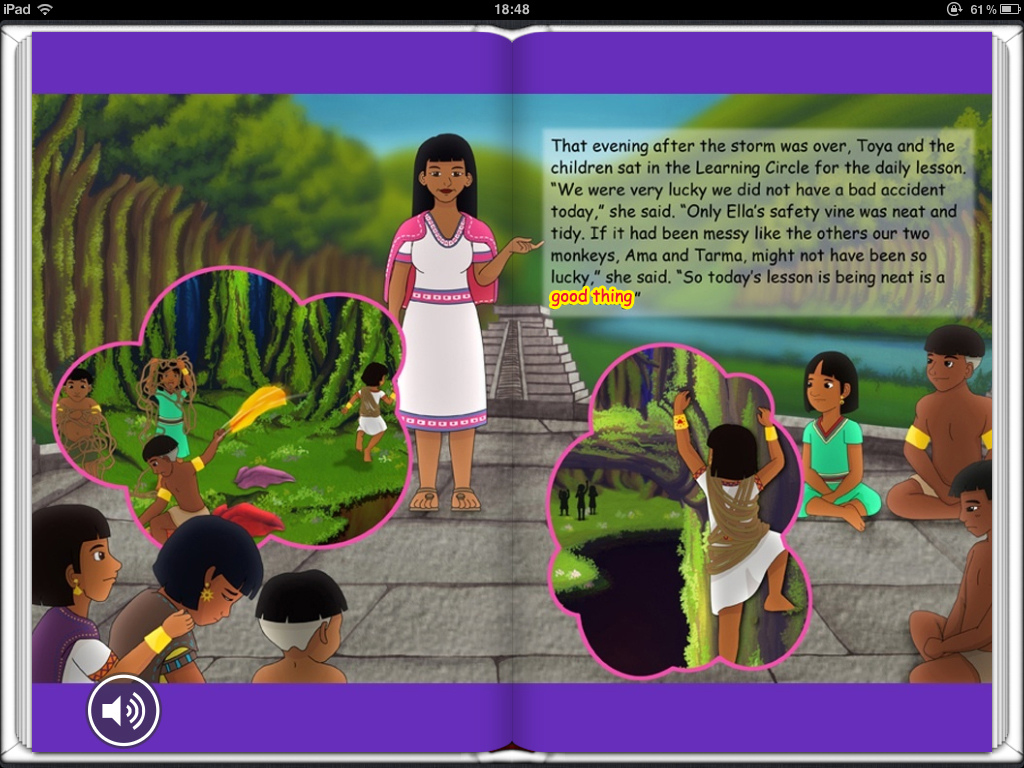The screenshot from an iPad features a page designed to mimic an open children’s book focused on cultural education, specifically Aztec or Mayan culture. A thin black bar across the top indicates it’s an iPad with the signal strength on the far left, the time displayed as 18:48 in the center, and the battery strength at 61% on the far right. 

In the book illustration, a female teacher dressed in traditional Aztec or Mayan attire, including a dress with a pink ribbon pattern and a pink shawl, is teaching a group of young, cross-legged children. Behind them is an ancient temple reminiscent of Aztec or Mayan architecture. The children have thought bubbles showing them playing in the forest.

There is a pale green text box with black writing next to the teacher, relaying a lesson. The text reads: "That evening after the storm was over, Toya and the children sat in the learning circle for the daily lesson. 'We were very lucky, we did not have a bad accident today,' she said. 'Only Ella’s safety vine was neat and tidy. If it had been messy, like the others, our two monkeys, Ama and Torma, might not have been so lucky,' she said. So today’s lesson is being neat is a good thing," with the last part highlighted in red with a golden border.

The environment depicted includes a stone or marble patio with trees flanking the left and possibly the right side, though partially obscured by the text box. A purple border frames the page, and a speaker icon is visible in the lower left corner, emphasizing that this is an interactive digital book on an iPad.